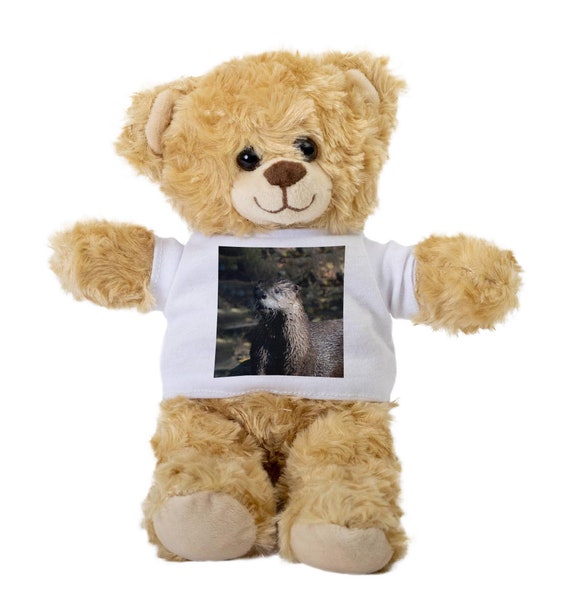The image depicts a small, cute, and fluffy teddy bear with light brown fur and beige accents on its feet and ears. The teddy bear has big, black button eyes, an embroidered brown nose, and a stitched smile, contributing to its happy and welcoming expression. Its arms are outstretched, as if ready to give a hug, and it appears to be either standing or propped up against an invisible support on a completely white background, suggesting it is for a product listing or advertisement.

The teddy bear is wearing a well-fitted, short-sleeved, white T-shirt. Prominently displayed in the middle of the shirt is a square image of an animal, which consensus suggests is likely an otter, although some descriptions mention it might be a beaver or even a cheetah. The animal in the image looks realistic, as if it is a photograph, and is portrayed in its natural habitat, complete with rocks, water, and trees in the background. This detail adds an interesting and possibly educational element to the bear's attire, making it both an adorable and potentially informative gift for a small child.